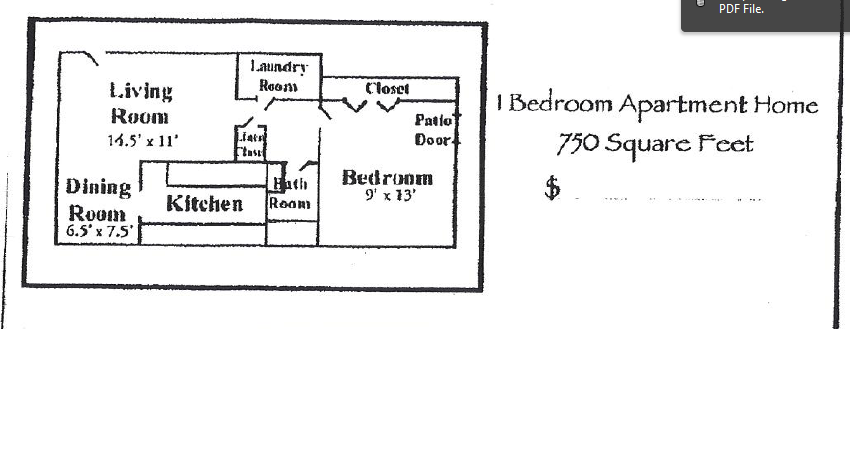This detailed black ink drawing illustrates the floor plan of a 750-square-foot, one-bedroom apartment home. The layout features a spacious living room measuring 16.5 by 11 feet, which seamlessly connects to a dining area of 6.5 by 7.5 feet. Adjacent to the dining room is the kitchen area, designed for convenient access. Next to the living room, a laundry room and a closet provide essential storage, with the bathroom entrance located directly opposite the laundry room. The bedroom, sized at 9 by 13 feet, includes a patio door, offering an outdoor extension of the living space. Additionally, the bedroom boasts a walk-in closet, enhancing the apartment's ample storage options.